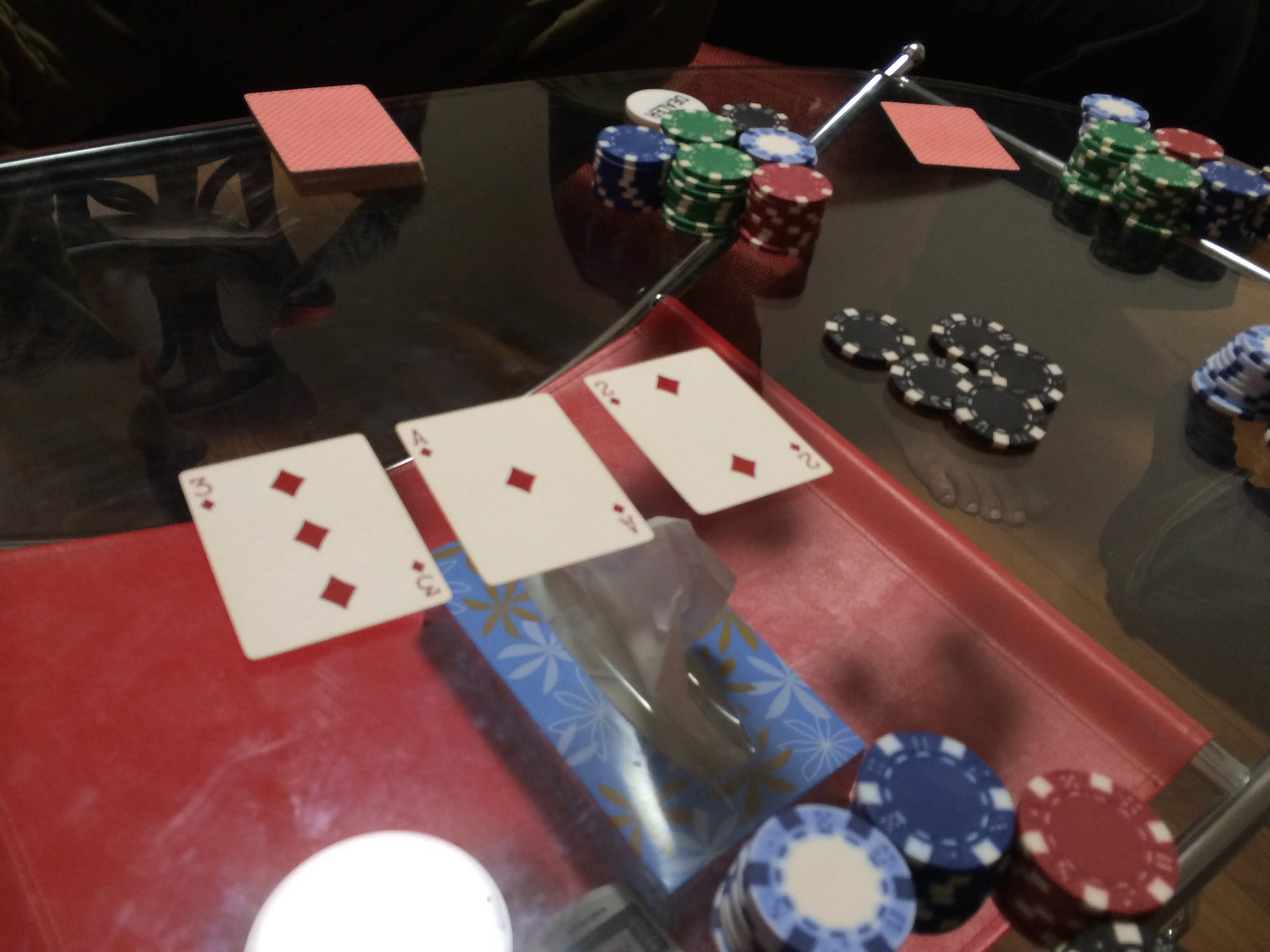In this image, a game of poker is in progress on a translucent glass table. At the center of the table, three cards are flipped face-up: the three of diamonds, the ace of diamonds, and the two of diamonds. Surrounding the face-down deck are several stacks of poker chips in various colors. Notably, the upper right-hand corner of the image features stacks of red, green, blue, light blue, and black chips, with five black chips prominently placed in the middle.

Underneath the glass table, a barefoot player is visible, alongside a floral box of Kleenex with a white tissue partially pulled out. On the right-hand side, through the translucent surface, a pant leg and a shoe of another participant can be seen, adding to the casual, yet competitive atmosphere of the game.